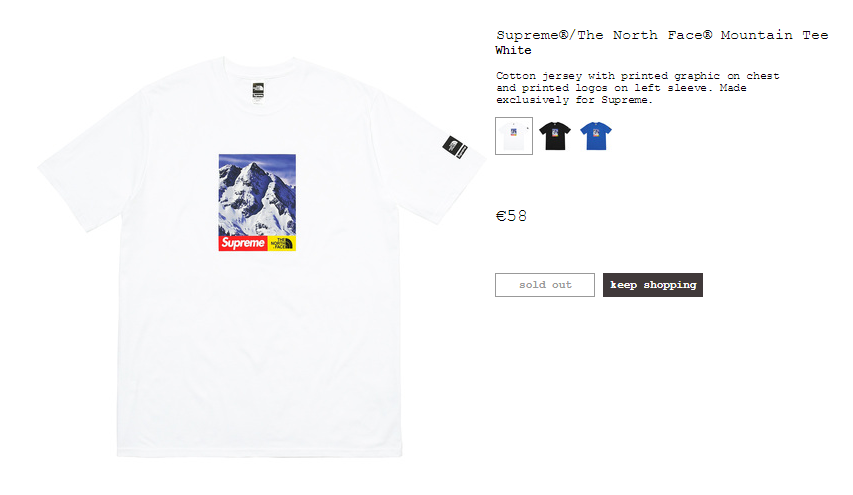A white cotton jersey t-shirt featuring a prominent, detailed printed graphic on the chest. The graphic showcases a snow-capped mountain under a blue-and-white sky, framed by two rectangles at the bottom. The left rectangle is predominantly red with the word "Supreme" in white lettering, while the right rectangle is yellow with "The North Face" phrase in bold black letters arranged in three rows (THE, NORTH, FACE), accompanied by the brand's iconic semi-circle logo.

On the right side of the chest graphic, the recognizable North Face logo is displayed, affirming the brand's identity without spelling out the full name. The left sleeve hosts additional branding with a black North Face logo featuring white text, situated next to the word "Supreme" in black font.

This exclusive collaboration piece, officially named "The North Face Mountain Tee," is designed exclusively for Supreme and is available in white, black, and blue color options. The design and color scheme may slightly vary but maintain the integrity of both brands' iconic elements.